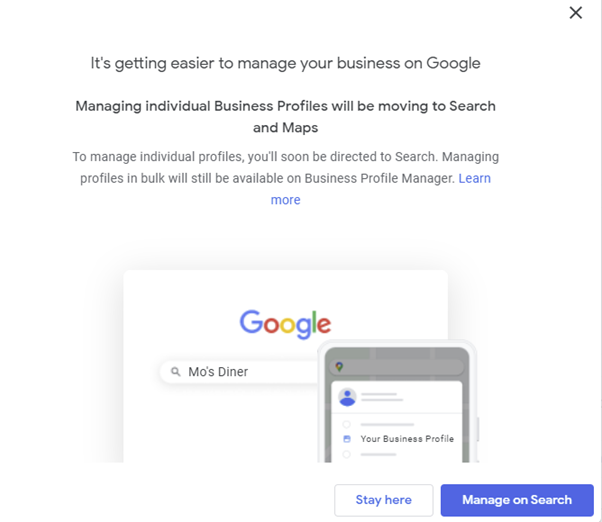The image features a Google interface update, illustrating the evolving process of managing business profiles. The screenshot reveals a prompt indicating that it will soon become easier to manage business profiles on Google, with individual profile management moving to Google Search and Maps. Users managing multiple profiles will continue to use the Business Profile Manager for bulk actions. 

The screen prominently displays the message: "Managing individual business profiles will be moving to search and maps. To manage individual profiles, you'll soon be directed to search. Managing profiles in bulk will still be available on Business Profile Manager," alongside a "Learn More" link in blue.

Below this message, the Google interface is shown with a search bar at the top, containing the text "Moe's Diner" in black. Adjacent to this, there is an image placeholder on a phone screen, indicated by two dots. The section titled "Your Business Profile" is highlighted in blue. The background of the phone's outer gray frame contrasts with the central interface elements.

At the bottom, two options are presented: "Stay here" and "Manage on search." The "Stay here" option appears in a white box with a gray circular border and blue text, while the "Manage on search" option is represented with white lettering inside a blue background and is currently selected.

The image demonstrates Google's new system for business profile management, detailing the transition process and showcasing the visual updates to the interface.